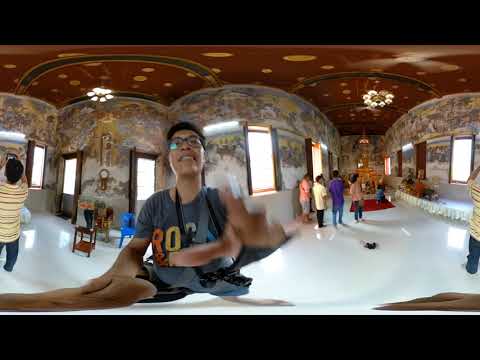A man with short black hair and glasses, wearing a blue rock t-shirt adorned with colorful lettering, is taking a selfie in a uniquely elaborate art installation that resembles a temple. The installation features intricately curved, bubbly, and ornate walls covered with paintings and murals that extend across every inch of the space. The floor is polished white, reflecting the vibrant and eclectic atmosphere around. The ceiling, painted red with white spots, hosts two flower-shaped chandeliers on either side. Behind the man, curved walls and windows gleam with lighting, casting a warm glow on the bustling crowd of around 10-15 people, many of whom are admiring the artwork or taking photos. A table adorned with flowers runs along one side of the installation. The man’s joyful expression captures the awe and wonder of this immersive and ornate environment.